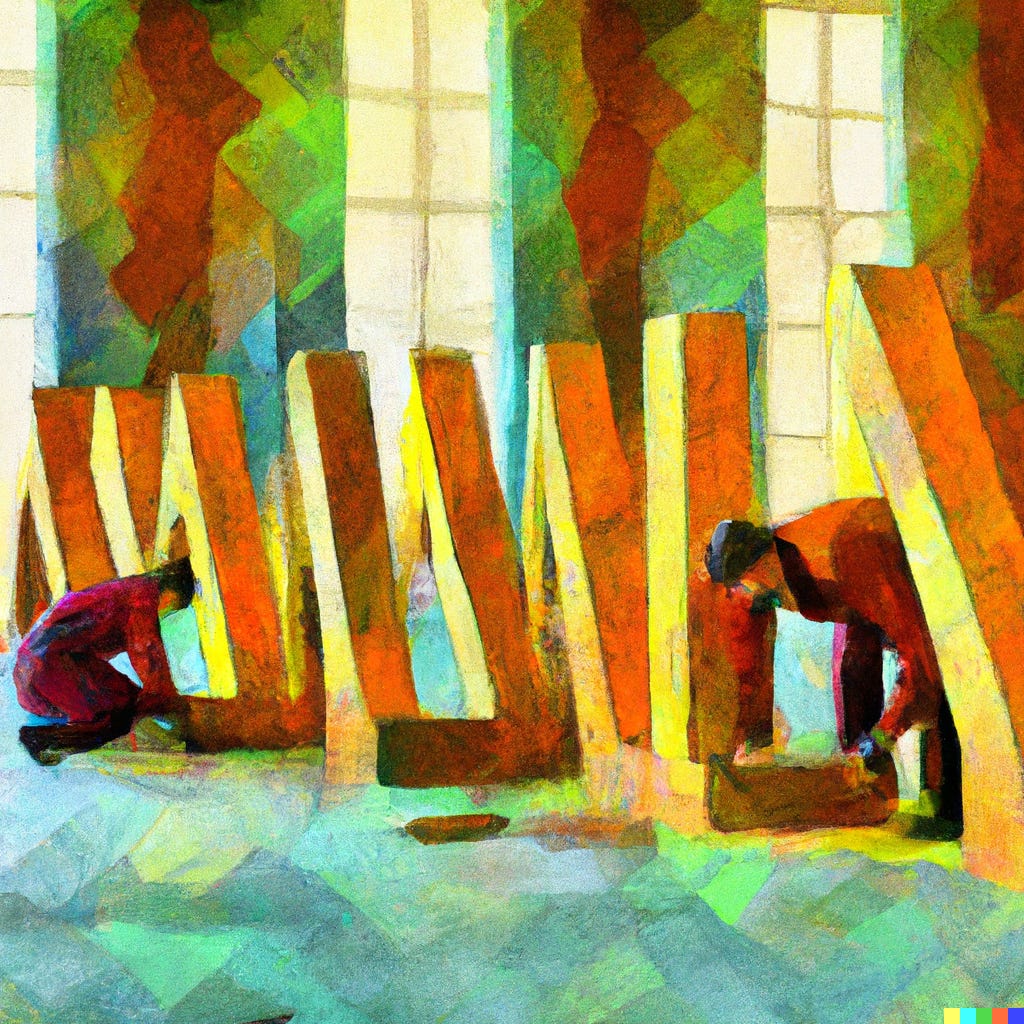The square, colorful illustration depicts an abstract scene, where two blurred figures in red jackets, black pants, and black hats are diligently working together to erect a sculpture made up of large, vertical columns shaped like letters. These letters reach about six feet in height and are painted a yellowish color with hints of tan or brown. The figures are bent over, seemingly hard at work, in a space richly detailed with vibrant hues. The floor beneath them features patches of neon green and aqua colors. Surrounding them, three tall, wall-to-ceiling panel windows framed by vertical columns allow yellow light to stream through, illuminating the area. These columns, decorated with a textured pattern of reddish orange, yellow, neon green, and blue squares, mirror a similar pattern found on the ground, save for the reddish orange. The entire scene is imbued with dynamic, artistic energy, showcased by the intricate interplay of colors and light streaming through the windows.